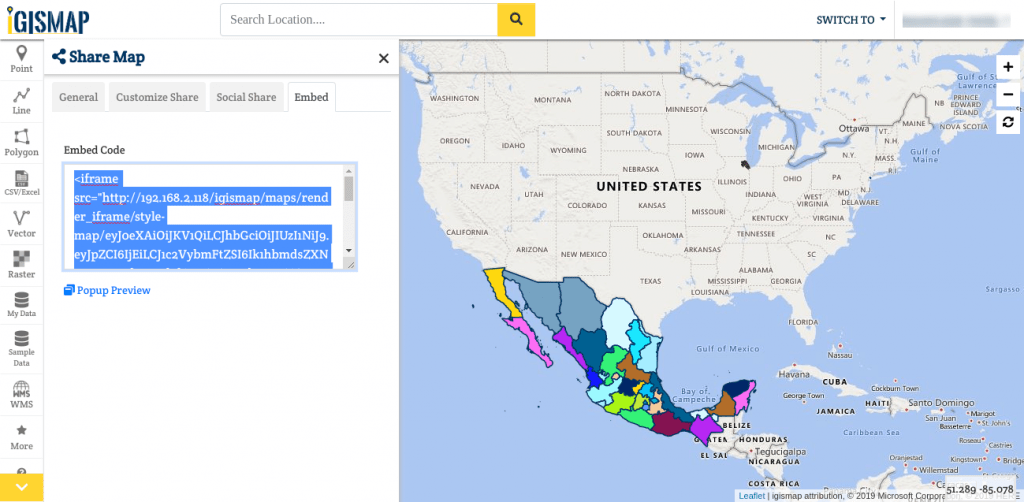A detailed screenshot showcasing a mapping interface is depicted. The main map area is predominantly shaded in blue and highlights the United States and Mexico. In this visualization, Mexico is further divided into individual states, each uniquely colored to distinguish them. 

A search bar is prominently positioned, featuring a yellow square with a black magnifying glass icon inside. This search bar is accompanied by a "Switch to" option, also styled in blue text. Below the map, there is a toolbar with several options: General, Customized, Share, Social Share, and Embed. The Embed option is currently selected, which is evident as it is highlighted in white. 

Within the selected Embed tab, an embed code box is displayed with its contents highlighted in blue, ready for copying. Additional features such as a pop-up preview button are colored in blue. The interface also provides versatile editing options listed as Point, Line, Polygon, CSV, Excel, Vector, Raster, My Data, Simple Data, WMS, and more. 

Lastly, a gray circular icon with a white question mark symbolizes help or information, and a yellow square containing a white down arrow signifies a dropdown menu or additional options.